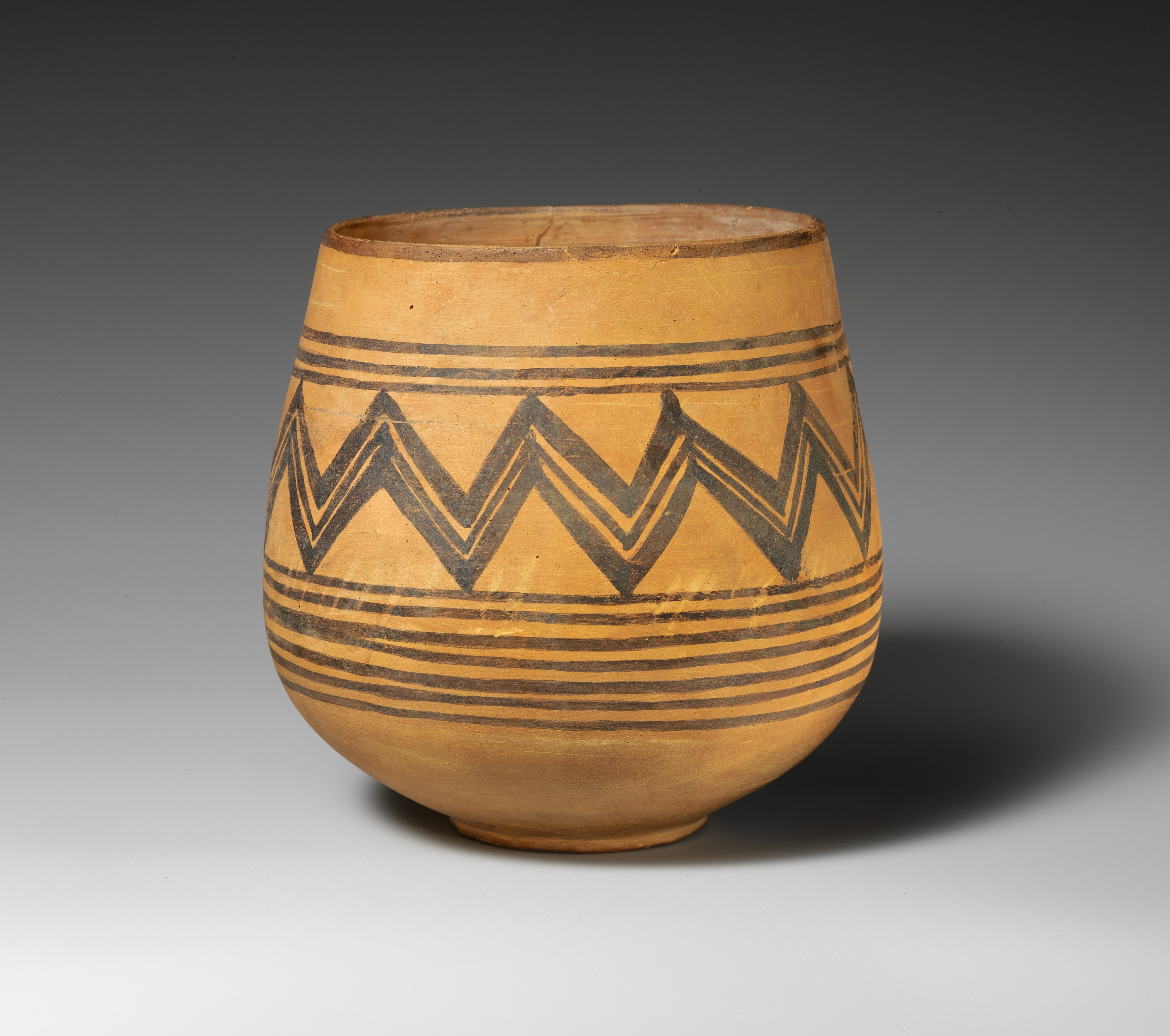The image depicts an ancient clay pot with a distinct orangish-yellowish, golden beige color, and a flat, slightly smaller base that expands and then narrows slightly towards the top, resembling a cup shape. The pot sits against a gradient background that transitions from white at the bottom to dark gray at the top. The surface of the pot features intricate designs: three dark brown or black lines encircle the top, followed by a chevron-like, squiggly square wave pattern reminiscent of Navajo or other North American Indigenous art. Below this, several thin, dark lines wrap around the pot, ranging from seven to eight in number, leading down to a bare bottom. The pot's exterior appears worn with etches, indentations, and scratches, suggesting its age and historical significance. A shadow is cast beneath, indicating its pedestal-like support, and the interior of the pot is a deeper brown than its exterior. The detailed craftsmanship hints that it was likely created with a spinning action, rather than solely by hand.